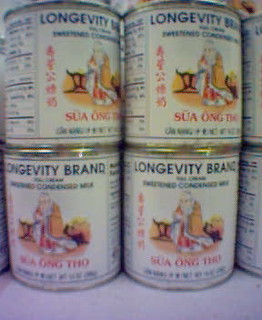The image features a stack of four cans of Longevity brand sweetened condensed milk, arranged in two rows of two. Each can sports a crisp white label with "Longevity brand sweetened condensed milk" prominently displayed in blue lettering. Dominating the front of each can is an illustration of an elderly Chinese man, depicted either sitting or kneeling, adorned in traditional Chinese robes. His attire includes orange sleeves, a red interior, and white trim, which adds a cultural richness to the presentation. Along the side of the can, red Chinese characters provide additional branding, accompanied by the text "S-U-A-O-N-G-T-H-O," also rendered in Chinese script. This neatly stacked arrangement appears to be part of a larger display, possibly on a store shelf.